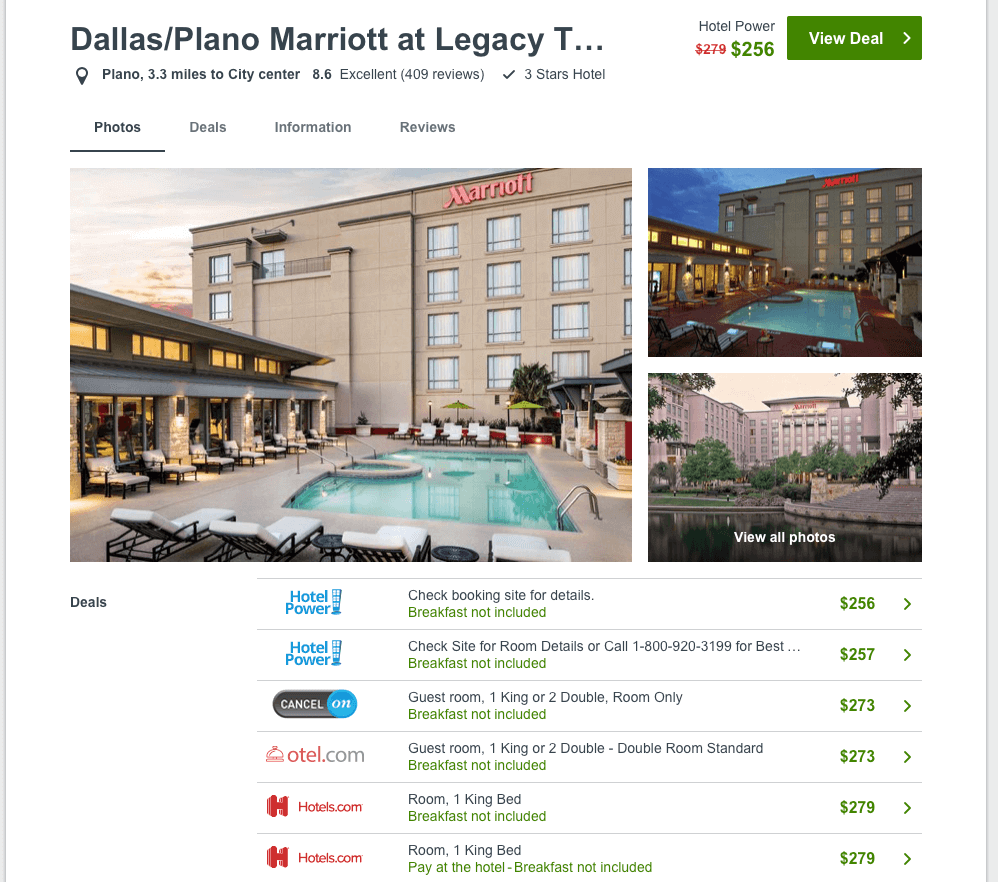This image showcases a webpage for the Dallas/Plano Marriott at Legacy Town Center, a three-star hotel located 3.3 miles from Plano's city center. The hotel has received a rating of 8.6 out of 10 based on 409 reviews. The page indicates that nightly rates range from $356 to $379 and provides a green button to view deals. The website features multiple photographs of the hotel, including images of its outdoor pool captured both during the day and at night, as well as the hotel's facade.

Beneath these pictures, there are several deal options listed. One indicates booking details with a mention that breakfast is not included. Another deal, labeled by 'hotel power', emphasizes an offer but again confirms that breakfast is excluded. Room options include a guest room with one king bed or two double beds. Pricing is displayed, with '273hotel.com' and 'anotherhotels.com' both listing rates at $279 in red. Green prices are accompanied by arrows on the right-hand side of the listings. Notably, none of the deals include breakfast.